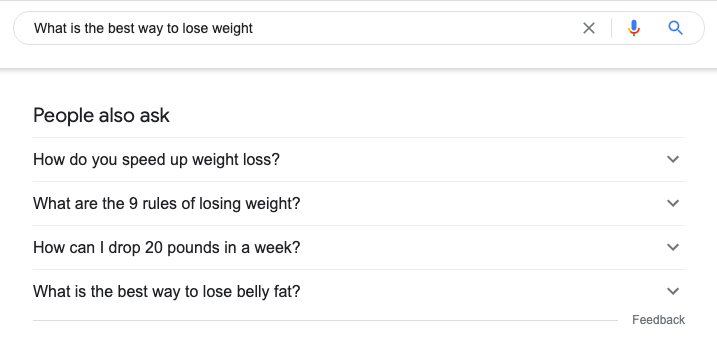The image depicts a screenshot of a Google search results page. At the top of the screen, the search query "what is the best way to lose weight" is prominently displayed, though it notably lacks a question mark at the end. The interface includes a red 'X' button on the far right to clear the query, a microphone icon for voice input, and a blue magnifying glass icon indicating that the search has been executed. The main content visible below the search bar is a "People also ask" section which lists four related questions: "How do you speed up weight loss?", "What are the nine rules of losing weight?", "How can I drop 20 pounds in a week?", and "What is the best way to lose belly fat?". Each question has a downward-facing arrow to its right, suggesting that clicking these arrows would reveal more detailed information. Finally, a "Feedback" link is visible at the bottom right corner of the screen. No specific website links or detailed answers are shown in this screenshot.